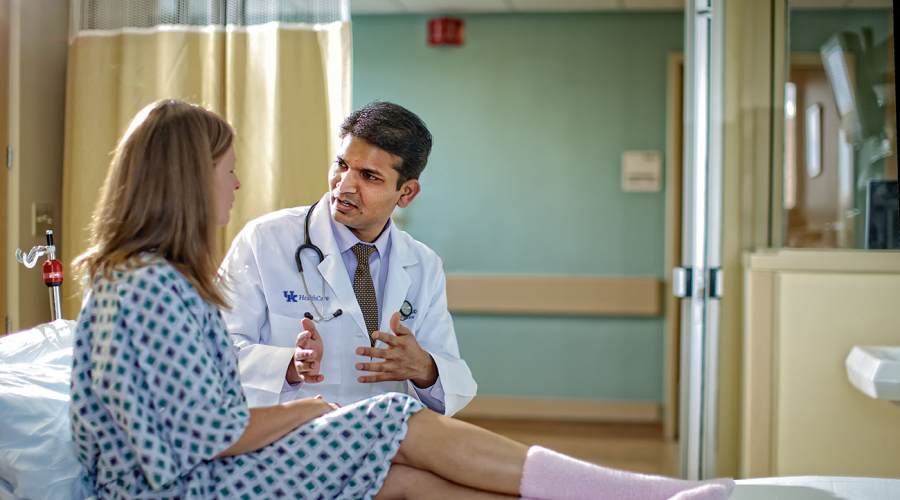In the photograph, you can see a hospital setting with light blue walls, an exit sign at the top, and a door with a room number beside it. There is a partially drawn privacy curtain visible as well. On a hospital bed is a middle-aged, slender woman with short sandy blonde hair, dressed in a checkered hospital gown with blue and black diamond shapes and pink socks. Sitting beside her is a young doctor, possibly of Indian or Asian ethnicity, who is wearing a white lab coat with a stethoscope around his neck. The doctor is gesturing with his hands as he explains something to the patient, who is listening intently. His face shows a serious expression as he tries to ensure that the patient understands what he is saying. The patient’s face is not visible as she is turned toward the doctor, making eye contact. The overall atmosphere suggests a focused discussion about her medical situation.